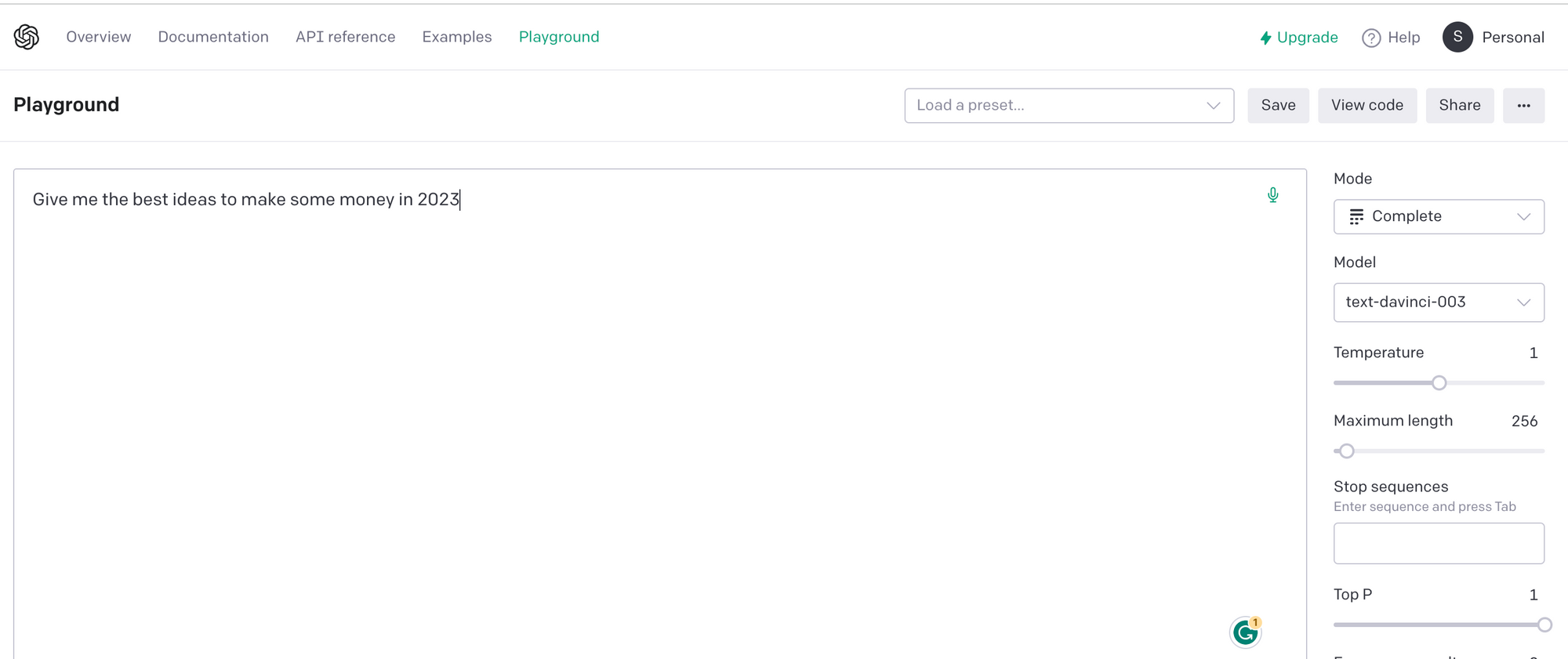A detailed screenshot of a black and white website interface with a few green accents. At the top left corner, there's a company icon resembling a pair of pinwheels. The navigation menu, which spans the top of the page, includes the options: Overview, Documentation, API Reference, Examples, and Playground, with Playground being highlighted in green. On the right side of the menu are three items: Upgrade, in green with a matching lightning bolt icon; Help, accompanied by a question mark; and Personal, denoted with a dollar sign.

Just below this menu, the word 'Playground' is prominently displayed in large, black text. Adjacent to it on the right, a set of buttons appear: Load a Preset, Save, View Code, Share, and an ellipsis leading to more options. Along the right-hand side of the screen, several parameters are listed, including Complete, Text, Davani003, Temperature, Maximum Length, Stop Sequences, and Top P. This interface appears to be part of a coding or AI platform, likely assisting users in configuring and running machine learning models.